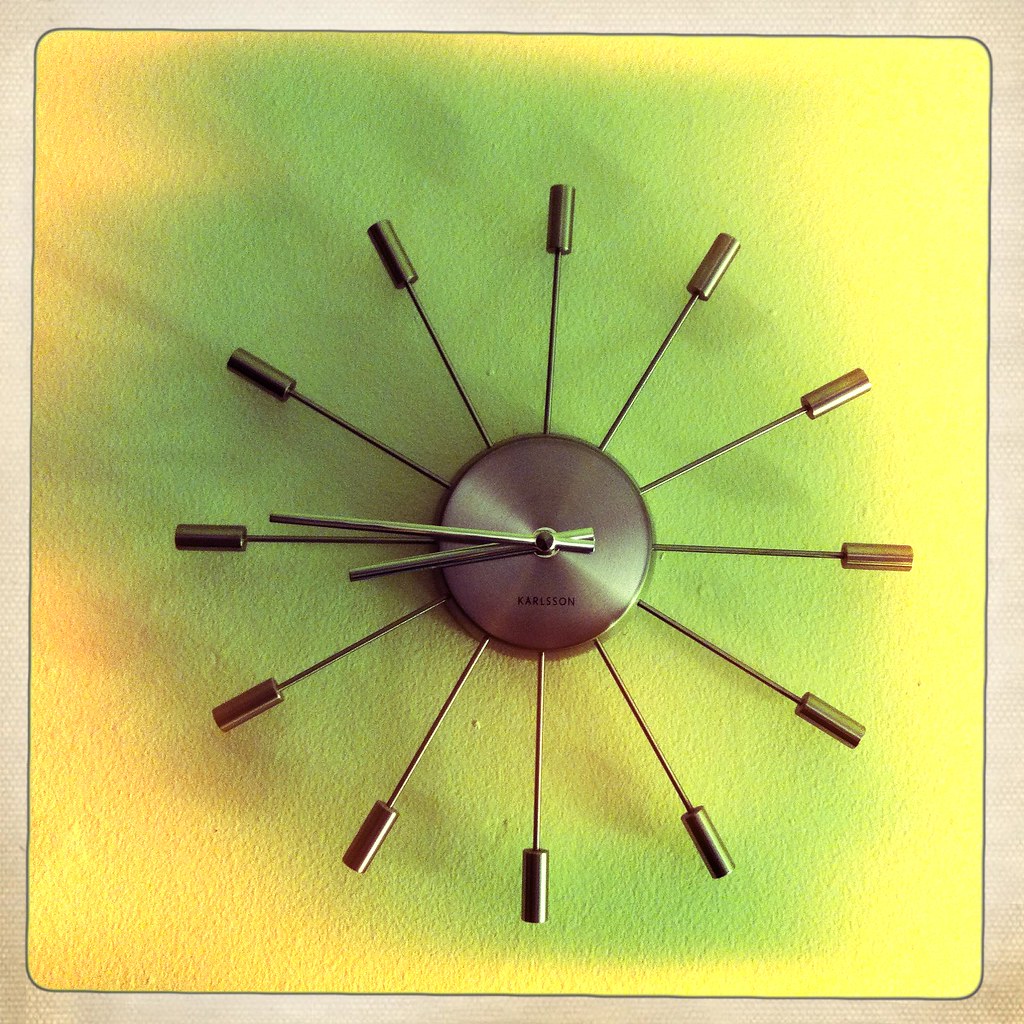This is a color photograph of a distinctive and abstract clock mounted on a wall. The clock features a minimalist design devoid of traditional numerical indicators. Instead, it has twelve thin metal spokes radiating from a central bronze circle, each tipped with a thick, cylindrical piece representing the hours. The clock hands, made of thick steel, are positioned towards the left, indicating the time as approximately 8:46. The branding on the clock is prominently displayed in black letters on the central circle, spelling "Karlsson." The background, a mix of yellow and green hues, further accentuates the clock's unique aesthetic, with the green color predominantly appearing directly behind the clock.